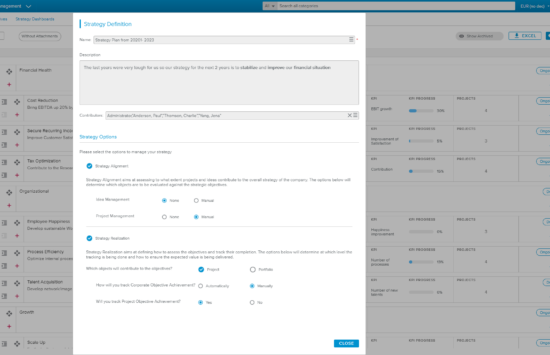This image is a very blurry screenshot of a website interface, obscuring most details. The top section displays a blue banner followed by a white search bar. Below this, the main content area shows a white page with the largest, most legible text on the top left reading "Stratology Definition" in blue. Underneath this heading are multiple sections: a narrow gray box, a larger gray box with a single line of black text, followed by a gray search bar. Further down, there is blue text on the left side and two circles with white check marks beside them. In the bottom right corner, there is an action button, though its label is unclear due to the image's blurriness.